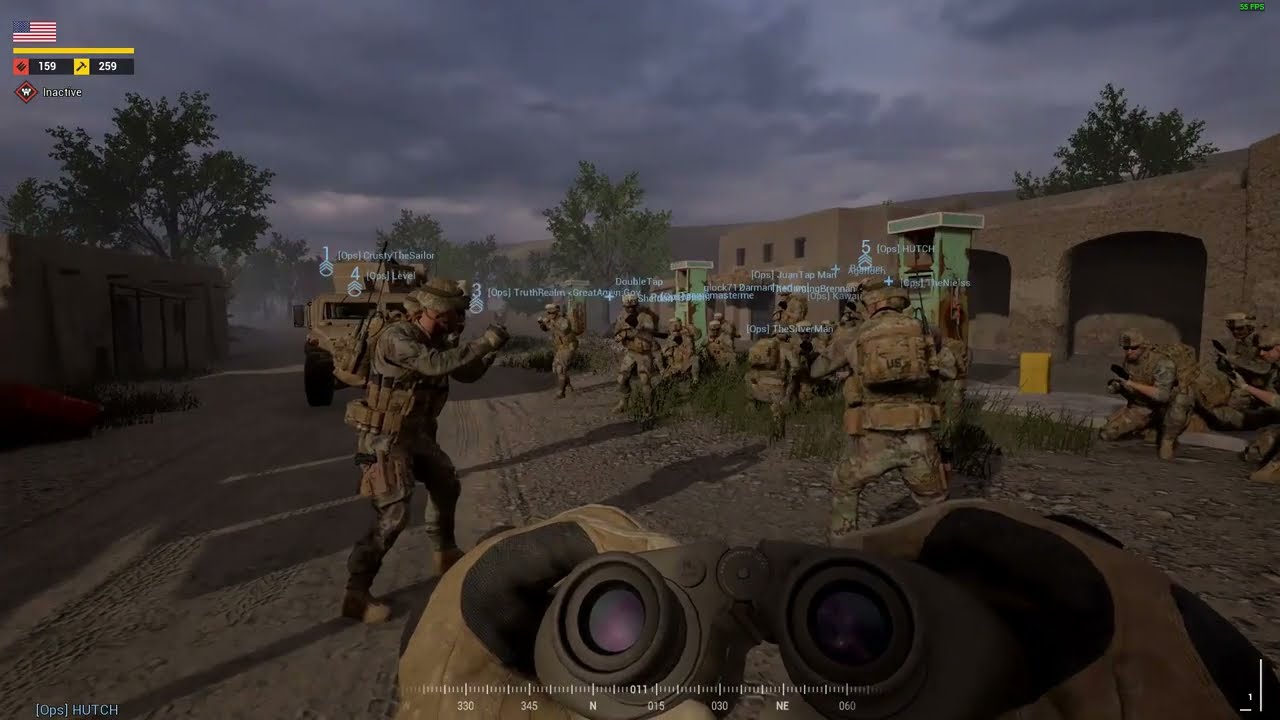The image depicts a first-person perspective screenshot from a military-themed video game, likely Call of Duty. The player character, identifiable through a pair of gloved hands holding black binoculars, stands in a desert-like environment. The leather gloves feature black palms and cream-colored exteriors. In the distance, we observe a group of soldiers kneeling and holding guns, outfitted in modern camouflage gear, including helmets and tan backpacks. They are split into two groups, each identified by colored lettering above them, likely indicating player names. The setting features a brown concrete or sandstone building with multiple entrances, resembling an abandoned garage or gas station. The scene is set against an overcast sky with some tree coverage and mountains in the background, creating an atmosphere of readiness and anticipation. Additionally, a compass visible in the player's interface shows they are facing east. The troops appear to be maintaining a low profile, possibly preparing for an imminent action.